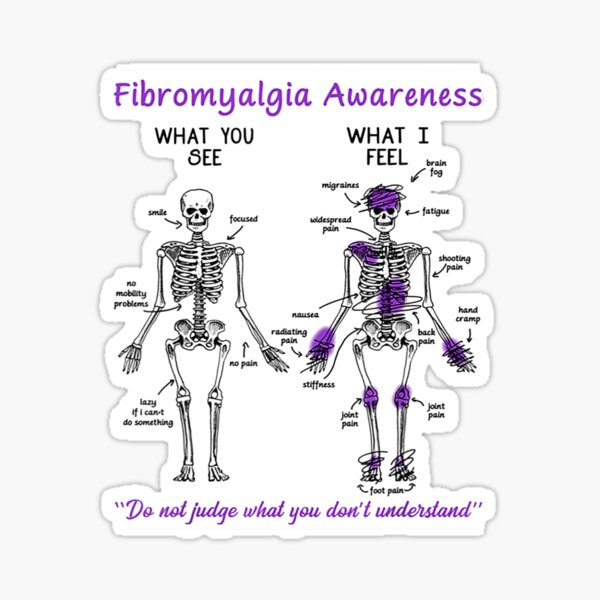The image, resembling an illustrated sticker or small magnet set against an off-white background, serves as a poignant illustration for fibromyalgia awareness. Dominated by a mostly black and white palette with strategic purple accents, the visual is titled "Fibromyalgia Awareness" in vibrant purple at the top. Central to the illustration are two skeletons side by side. The skeleton on the left, labeled "What You See," appears normal with labels highlighting typical perceptions like "Smile," "Focused," "No Mobility Problems," and "No Pain." In stark contrast, the skeleton on the right, under the label "What I Feel," is marked with purple blotches at various points, symbolizing areas of pain and discomfort such as the wrist, knees, chest, right shoulder, and forehead. These purple spots indicate conditions like "Joint Pain," "Foot Pain," "Migraine," "Fatigue," and "Brain Fog." Beneath the skeletons, a powerful message in purple letters insists, "Do Not Judge What You Don't Understand," inviting viewers to empathize with the unseen challenges faced by those with fibromyalgia.